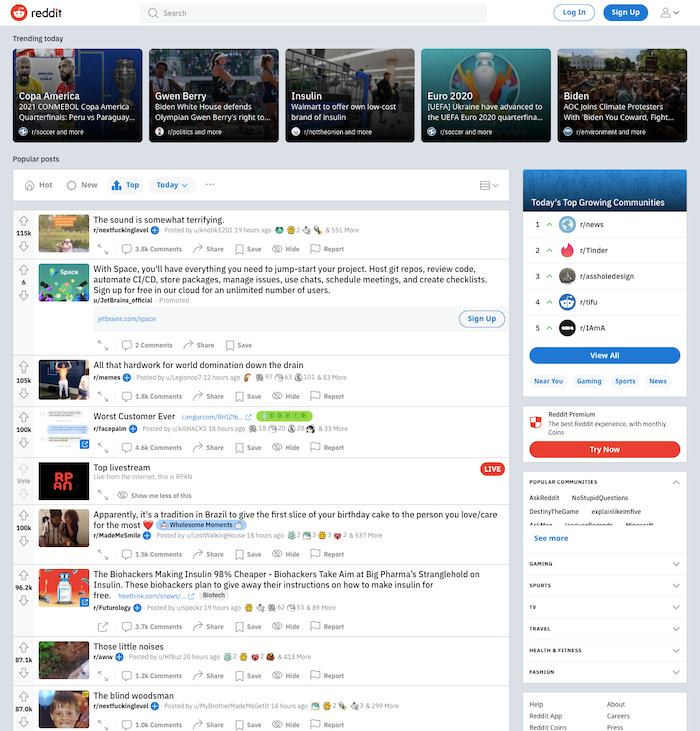Here's a cleaned-up and detailed caption for the described image:

"The webpage in the image is from Reddit. The iconic red circle with a white alien logo prominently displays 'reddit' in red and 'black' in the upper left corner. At the top of the page, there is a gray search bar accompanied by 'Log In' and 'Sign Up' options, as well as a generic profile picture with a drop-down arrow, placed on the right side. Below the navigation bar, a 'Trending Today' section features images and headlines. Highlights include a picture of Copa America, Gwen Berry, two women with a headline about Walmart offering a new low-cost brand of insulin, Euro 2020, and an image of President Biden with climate protesters. The webpage's body is filled with text and information, listing popular posts. Headlines such as 'The sound of some...is somewhat terrifying' and 'All the hardware for world domination down the drain' can be seen, reflecting current topics. On the right side, a blue bar highlights today's 'Top Growing Communities' with icons and names listed below. A button with 'View All' allows further exploration. Additionally, there's a section for Reddit Premium, inviting users to 'Try Now' via a red button, with popular communities and their details listed underneath."